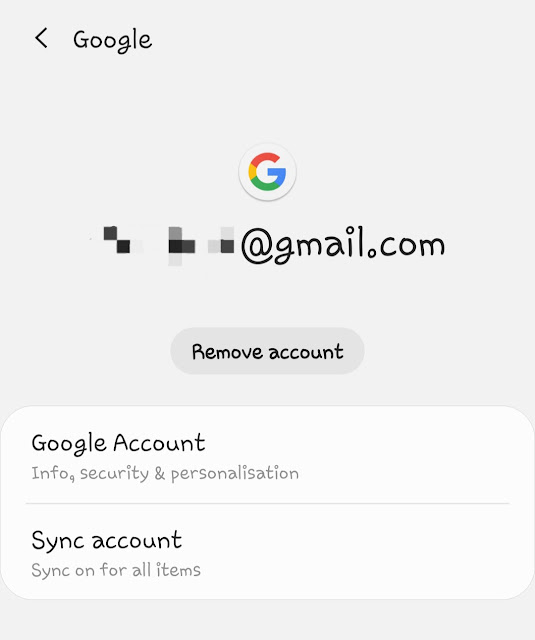This image captures a distinctive visual representation of a Gmail account interface. Set against a light gray, almost off-white background, the scene is dominated by Google's signature branding. At the top, the word "Google" is prominently displayed in black font, suggesting a unique or less commonly used typeface that mimics handwritten text, giving the interface a homemade, personal feel.

A left-pointing arrow is positioned near the top left corner, indicating a back navigation option. Central to the composition is the iconic Google "G," depicted in a vibrant array of rainbow colors—orange, yellow, green, and blue—immediately drawing the viewer's attention.

Beneath this colorful "G," an email address is presented, partially obscured for privacy, ending with "@gmail.com." Below the email, there is an actionable option labeled "Remove account."

The lower section of the interface provides additional account management options, listed as "Google account, info, security, and personalization," followed by "Sync account" with a status note "sync on for all items."

Overall, the interface conveys a blend of familiarity and uniqueness, primarily due to its unusual, handwritten-style font, which adds a personal, almost nostalgic touch to the otherwise modern digital setting.